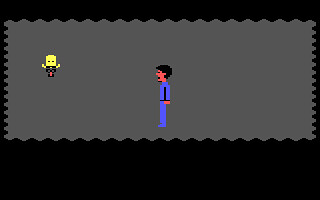This image is a screenshot from a pixel art game, featuring a striking contrast between the elements. The background is entirely black, making the main subjects stand out. In the center, there's a smaller, horizontally-oriented rectangle that spans the entire width of the image but is noticeably shorter in height. This rectangle has unique, wavy edges, adding a decorative border to the scene within.

Inside the rectangle, the interior is filled with a flat gray color. Dominating this space is a side-view pixel character, standing still. The character is depicted with a blue jumpsuit, arms resting naturally at their sides. The individual has a pinkish-peach complexion and short, black hair. Their facial expression, highlighted by a slightly open mouth, suggests curiosity or surprise.

To the left of this character is a small, floating creature. This whimsical being features a yellow head and similarly colored arms extended outward, contrasted by a tiny black body. The creature is airborne, defying gravity, and appears to be the focal point of the character's gaze. The pixel man is facing to the left, his attention completely captured by this odd, levitating figure.